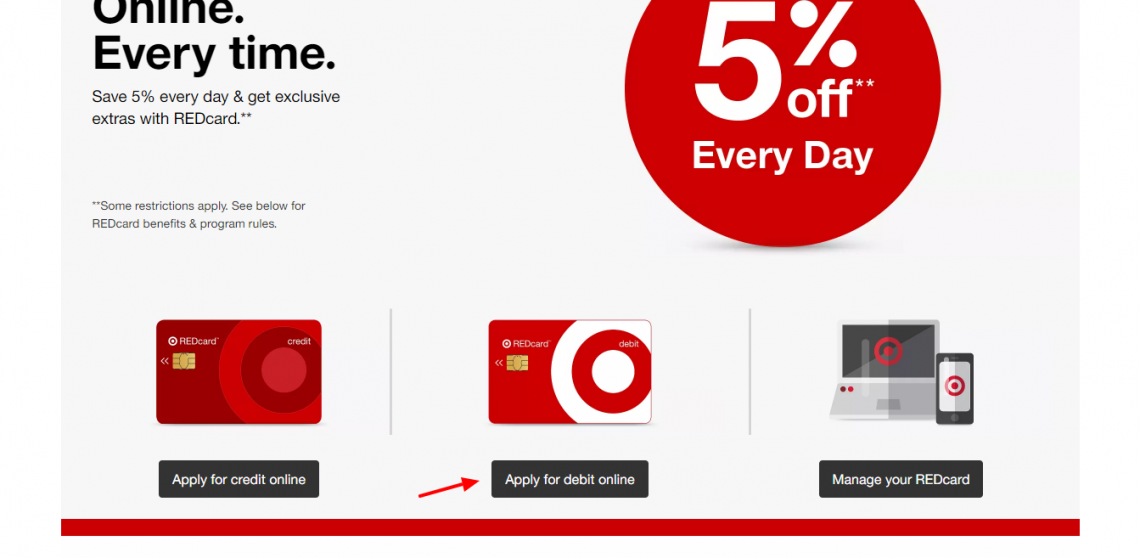This image appears to be an advertisement for Target, although the logo is not explicitly mentioned. The recognizable Target symbol, a red circle surrounded by a white circle, which is then surrounded by another red circle, is present.

The advertisement text, slightly cut off at the top, states, "Online every time." It also highlights that customers can "Save 5% every day and get exclusive extras with REDcard," with "RED" prominently written in all capital letters. To the right, a large red circle features the text "5% off every day" in white font. 

Next to the REDcard, there is a note about terms: "Some restrictions apply, see below for REDcard benefits and program rules." The ad showcases two types of REDcards. One card, more burgundy with red accents, instructs potential applicants to "Apply for credit online." Another version, predominantly white with red highlights, also encourages users to "Apply for credit online." Additionally, there is an image of a cell phone and a computer with the message "Manage your REDcard."

Overall, the advertisement emphasizes the benefits and ease of applying for and managing a Target REDcard online, while constantly reminding viewers of the 5% savings and exclusivity it offers.